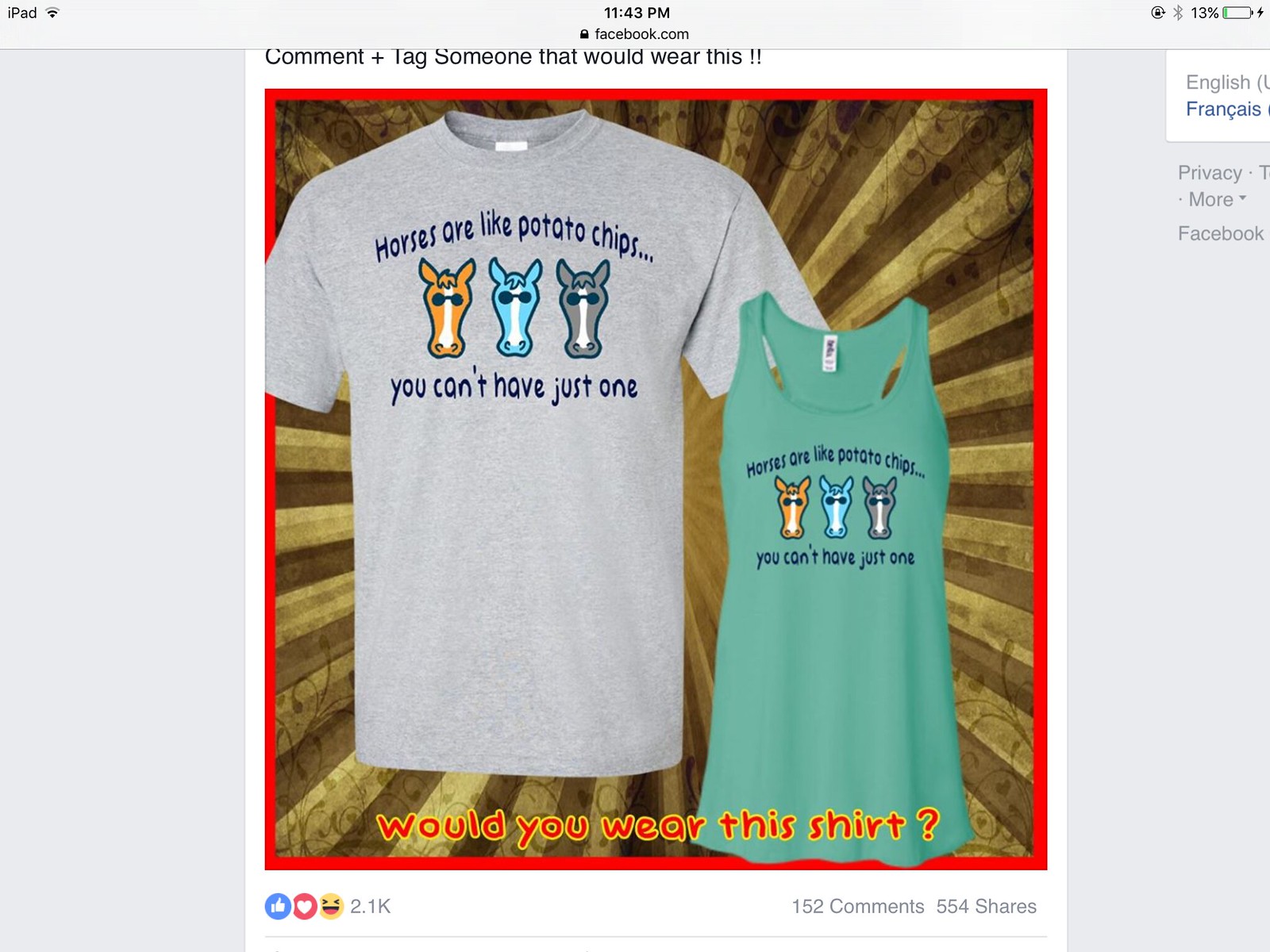This detailed image captures a screenshot, presumably taken from a Facebook post using an iPad, indicated by the "iPad" label, Wi-Fi symbol, and a 13% battery icon on the screen displaying a green charging sign. It is 11:43 p.m., and various indicators show Bluetooth is on, and the portrait view lock is enabled. The post features an eye-catching design of two shirts against a beige background with a darker brown sunburst effect. One shirt is light gray, and the other is a light green tank top, both displaying the phrase, "Horses are like potato chips, you can't have just one." Each shirt shows three horse heads from left to right: one orange, one light blue, and one gray—all wearing sunglasses. At the top of the image, a prompt advises, "Comment plus tag someone that will wear this," and at the bottom, a red text queries, "Would you wear this shirt?"